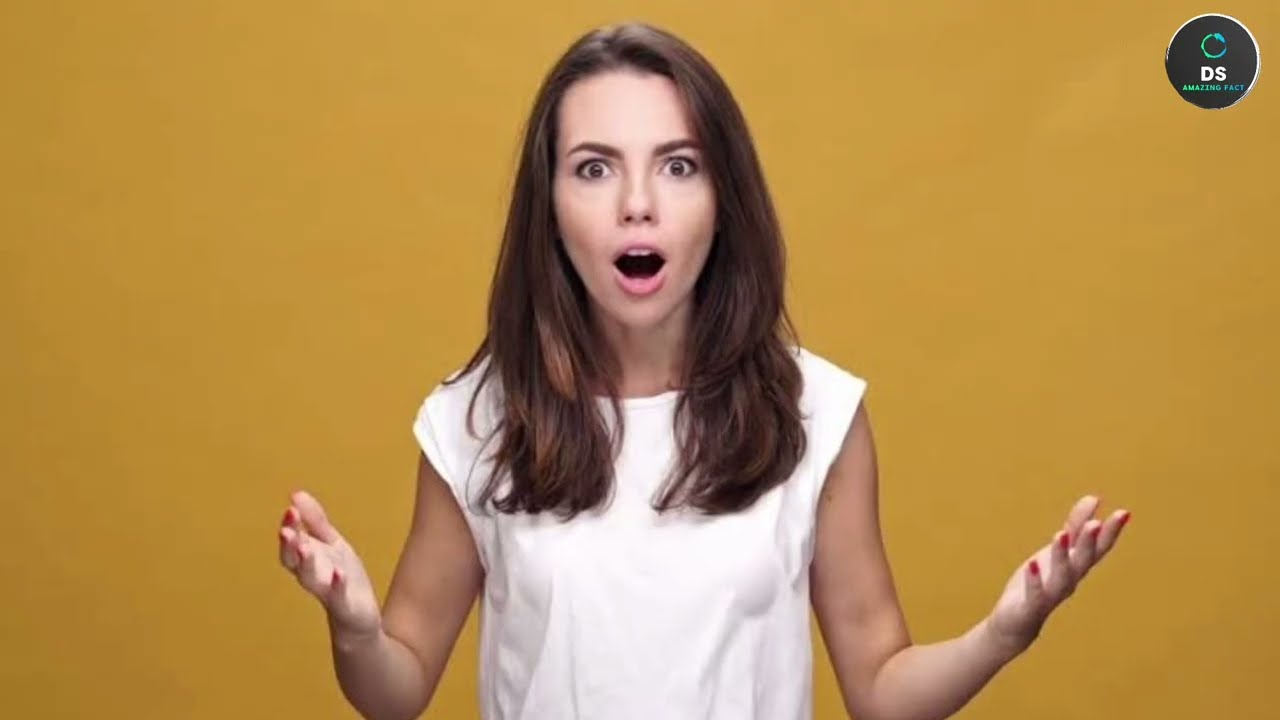The image depicts a young Caucasian woman with long, shoulder-length brown hair that is parted slightly to her right. She stands in front of an abstract, mustard-yellow to brownish-gold background with slight variations in color. At the top right corner, there is a circular emblem with a dark interior and a white border, containing the white capital letters "DS." Below this emblem is additional text, though it's not fully legible. The woman, wearing a white tank top that resembles a sleeveless t-shirt, displays an expression of manufactured surprise suited for a stock photo. Her mouth is wide open, revealing her top front teeth, and her eyes are agape with eyebrows raised. Her arms are outstretched in front of her with palms up, showcasing red or dark pink fingernails that match her light pink lipstick. The overall scene suggests a moment of exaggerated astonishment.